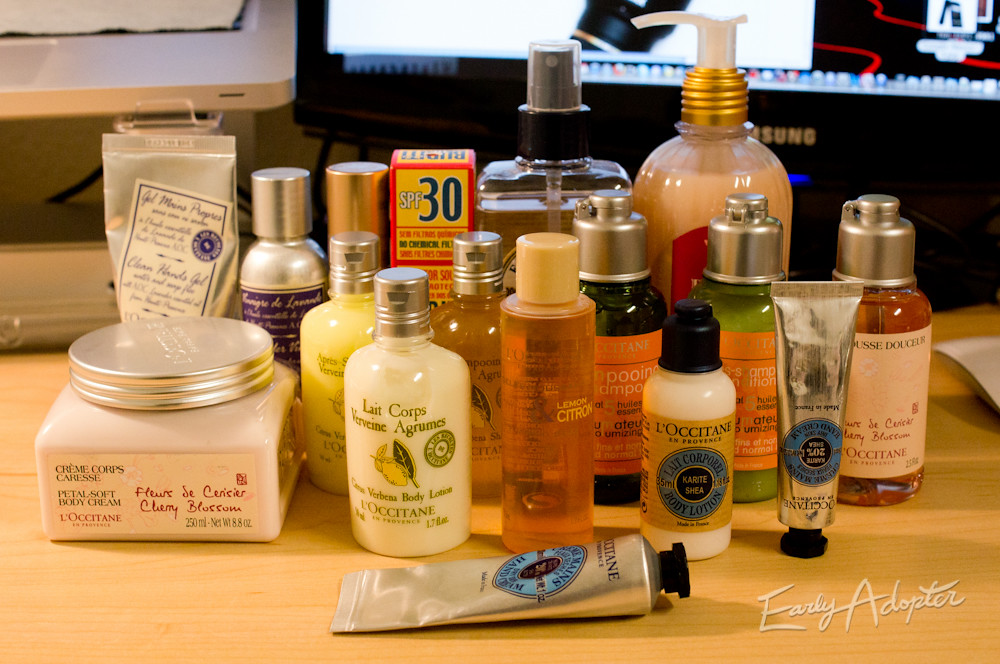This image features a sleek, light wood desk or table. Dominating the background is a Samsung screen, which could either be a computer monitor or a small television. To the left of this screen stands a mysterious white electronic device whose function is not entirely clear. The table is adorned with an array of skincare products, many of which appear to be from the L'Occitane brand, recognizable by its distinctive French labeling. Among the collection, there are jars, tubes, and bottles, including a large bottle equipped with a pump dispenser. Notably, there's also a bottle of sunscreen labeled SPF 30 amidst the assortment. This detailed display typically includes creams, lotions, and sprays, reflecting a comprehensive skincare routine.